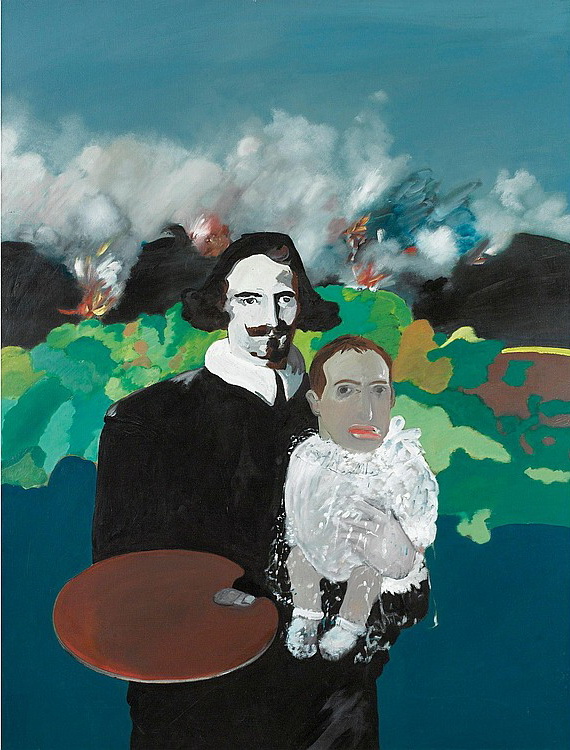This painting possesses a surreal and abstract quality, merging various colors and elements into a striking composition. The backdrop is a chaotic blend of smeared blues and greens, overlaid with white streaks, and populated by indistinguishable shapes reminiscent of wings or feathers in shades of pink and white, as well as reaching clouds. Dominating the foreground is a lone figure strikingly clad in black with a prominent white collar, echoing the attire of a 19th-century musketeer or Shakespearean figure. He has distinct, off-to-the-side black hair and a handlebar mustache, complete with a black soul patch under his lip. 

In his left hand, this character holds a peculiar baby dressed in a white chiffon outfit with exposed legs and socks, but bearing the incongruous adult visage of a man, strikingly hinted to resemble Mark Zuckerberg. The baby’s abstract face is accentuated with exaggerated features such as big lips and dark eyes. In the character's right hand, there is a brown artist's palette dotted with paint. The scene around them includes an explosion of colorful chaos, including elements reminiscent of erupting volcanoes with orange hues and smoke, alluding to a fantastical, surreal world between reality and imagination.